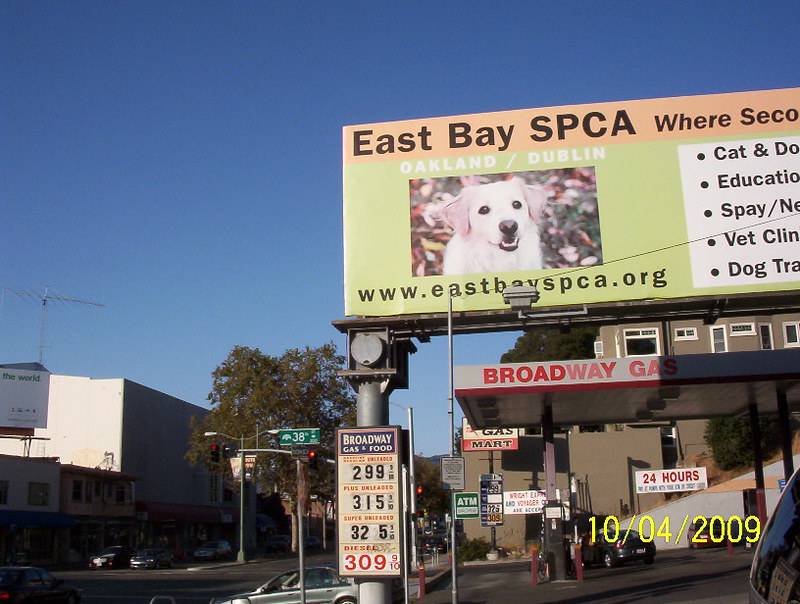This is a detailed photo of a bustling city street scene captured on October 4, 2009, prominently featuring a gas station on the lower right corner. The gas station's canopy, topped with red letters reading "Broadway Gas," shelters the fueling area where a car is being filled up. Above this, a large, eye-catching yellow billboard is supported by cylindrical posts, promoting the East Bay SPCA with black letters on a light orange backdrop and a website link, www.eastbayspca.org. The billboard also showcases a photo of a white labrador-like dog standing on leafy ground, with a dark black nose, slightly open mouth showing its teeth, and dark eyes against a beautifully clear blue sky.

The scene includes additional details such as a metal pillar supporting both the billboard and a smaller gas station sign indicating "Broadway Gas and Food." Gas prices displayed are $2.99, $3.15 for premium, and $3.09 for diesel, a nostalgic nod to the era. A street sign for 38th Street confirms the location, and the road is dotted with cars, buildings, and a prominent tree on the left. Stores line the street behind the gas station, adding to the urban environment's bustling yet orderly feel. The sky is strikingly blue, enhancing the clarity and vibrancy of the scene.